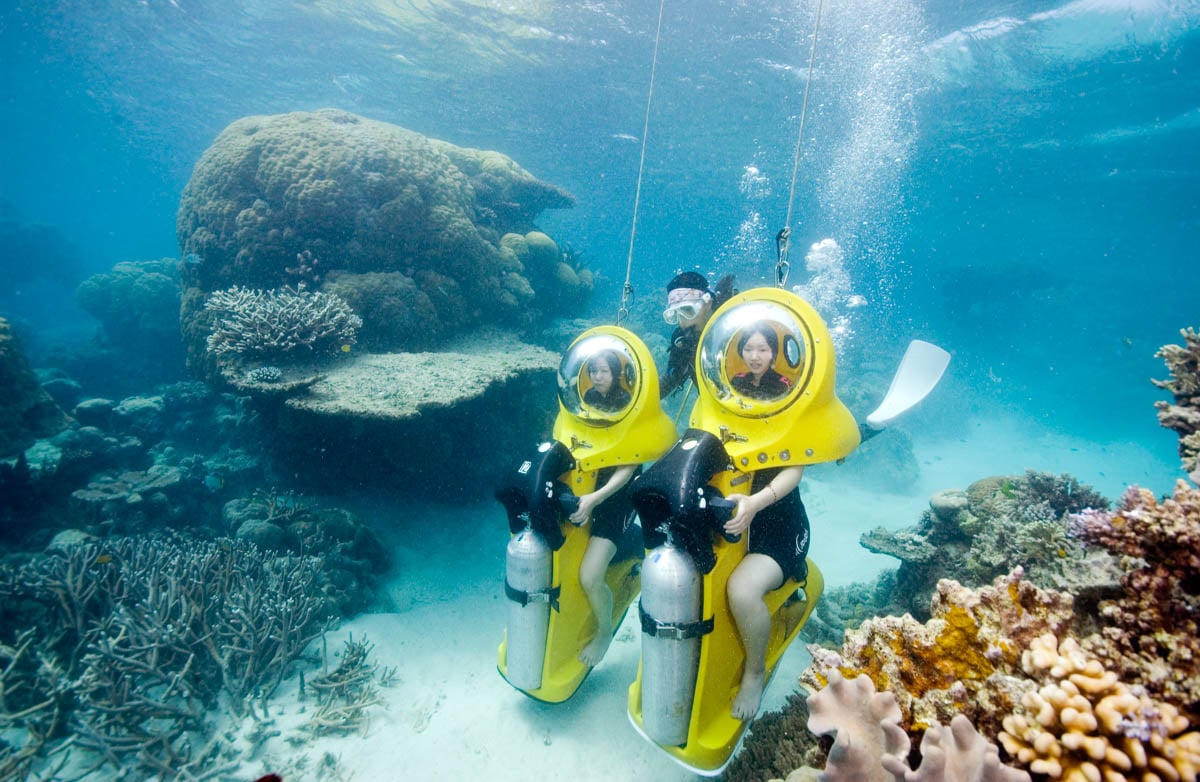In this underwater photograph taken in the ocean, two women are seated on yellow, scooter-like contraptions navigating a coral reef with a white sandy bottom. These unique vehicles resemble water mopeds, each equipped with an oxygen tank attached to the front, handlebars, and a large, dome-shaped helmet that encloses the women's heads, allowing them to breathe. The helmets create an astronaut-like appearance, making their heads look small and somewhat contorted due to the curvature of the glass. The women, dressed in black swim outfits comprising shorts and shirts, are positioned side by side in the center of the image, with the scooters connected to cables extending upwards, suggesting a shallow depth.

A scuba diver dressed in standard gear, including a bandana and white goggles, can be seen behind the women, likely ensuring their safety as they explore. The coral reef itself is depicted with vivid detail—featuring a variety of corals, including brownish "popcorn shrimp"-like formations and denser, furball-like structures, along with branched corals. The overall scene captures a vibrant underwater world and offers a unique perspective on interacting with a coral reef environment.